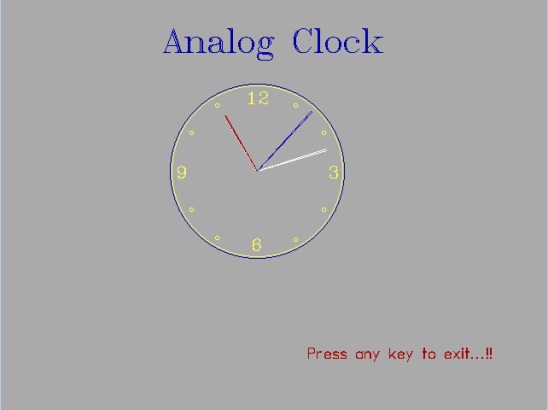The image depicts an analog clock set against a solid gray square background. At the top center of the image, in blue serif font, is the title "Analog Clock" with capitalized letters. Below this text, a blue circular clock face is prominently displayed. The clock features only the primary numbers 12, 3, 6, and 9 in a light yellow color, with smaller circles marking the other hour positions. The minute hand, colored blue, is positioned between the 1 and 2 markers, while the hour hand in white points between the 2 and 3 markers. The red second hand points directly at the 11. In the lower right corner of the image, there is red text that reads, "Press any key to exit..." followed by two exclamation marks.